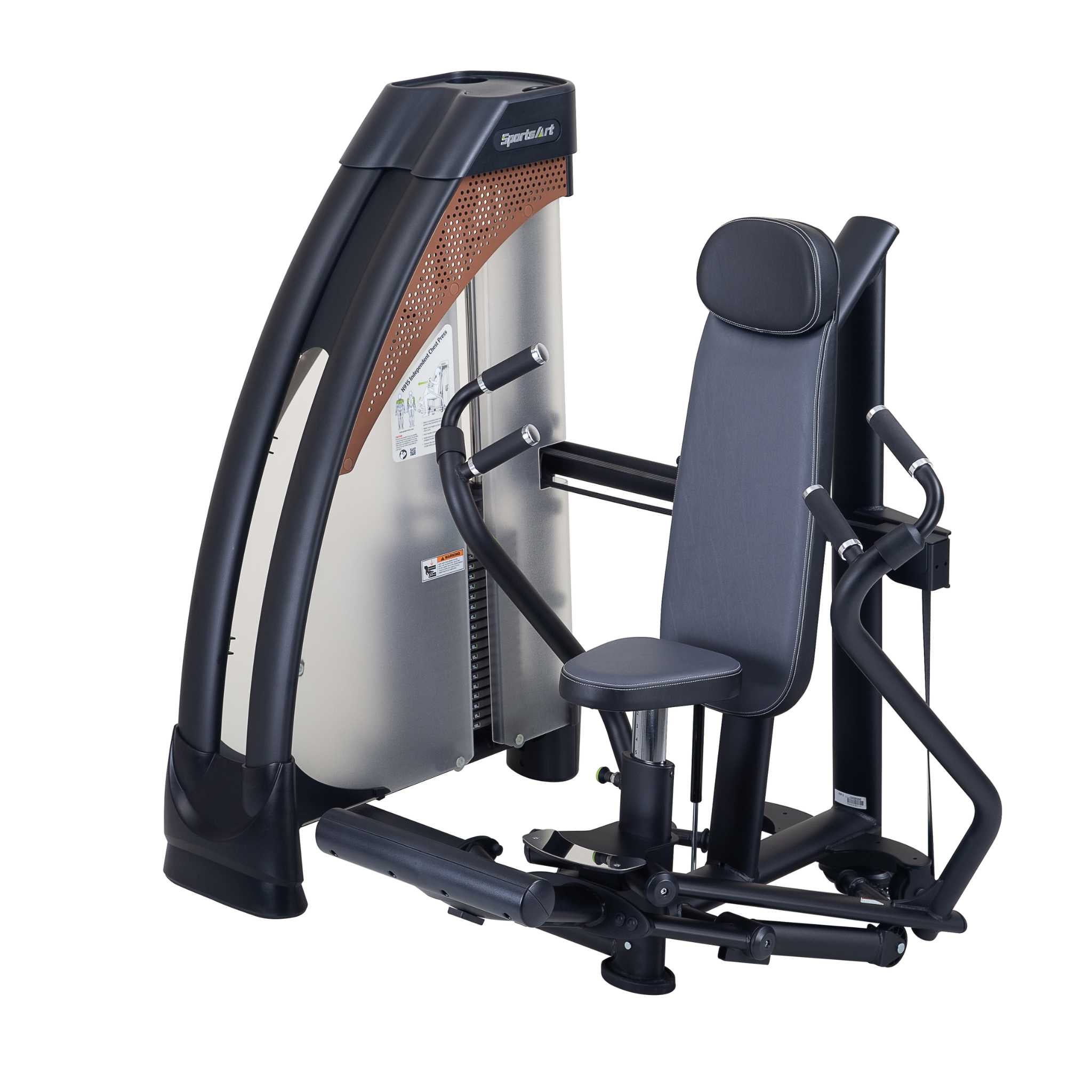The image portrays an outdated, clunky workout machine, primarily made of black, dark gray, and stainless steel materials with chrome accents. On the right side of the machine, a brown metal accent indicates the main component housing the weights, visible behind a plastic cover. The left side features an upright mechanism with black legs supporting it. This machine seems designed for seated arm exercises, equipped with a gray and black chair and dual-position handles at chest level, allowing users to either push or pull to lift weights. The setup suggests a resemblance to a rowing machine, specifically engineered to target arm strength through adjustable hand grips and positions. A SportsArt logo labels the equipment, reinforcing its identity as a fitness apparatus.